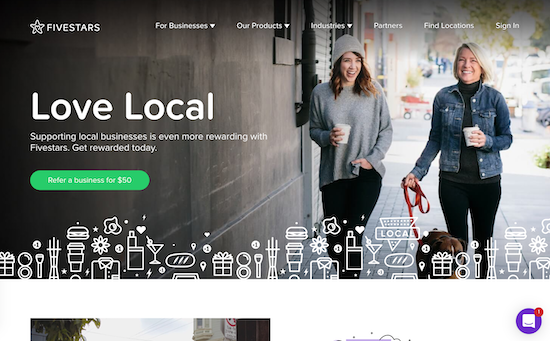The image showcases the top portion of a website, approximately 50% wider than it is tall. Dominating around 75% of the viewing area from the top is the main banner featuring an outdoor urban scene. The left half of the image captures a stark cement wall of a building, transitioning into a light gray steel garage door designed for vehicle entry. 

Along the right side of the building, two women are walking down the sidewalk, seemingly in their thirties or forties, both are Caucasian, smiling, and laughing. The woman on the left has brown hair while the woman on the right has blonde hair.

Overlaying the banner on the left-hand side, about a third of the way down, is prominent white text stating "Love Local." Below this, in a smaller white font aligned to the left, the text reads, "Supporting local businesses is even more rewarding with FiveStars. Get rewarded today." Directly underneath is a noticeable green button with white text that reads, "Refer a business for $50."

In the upper left-hand corner of the entire page, the FiveStars logo is displayed, consisting of the words "FiveStars" alongside an icon of a star.